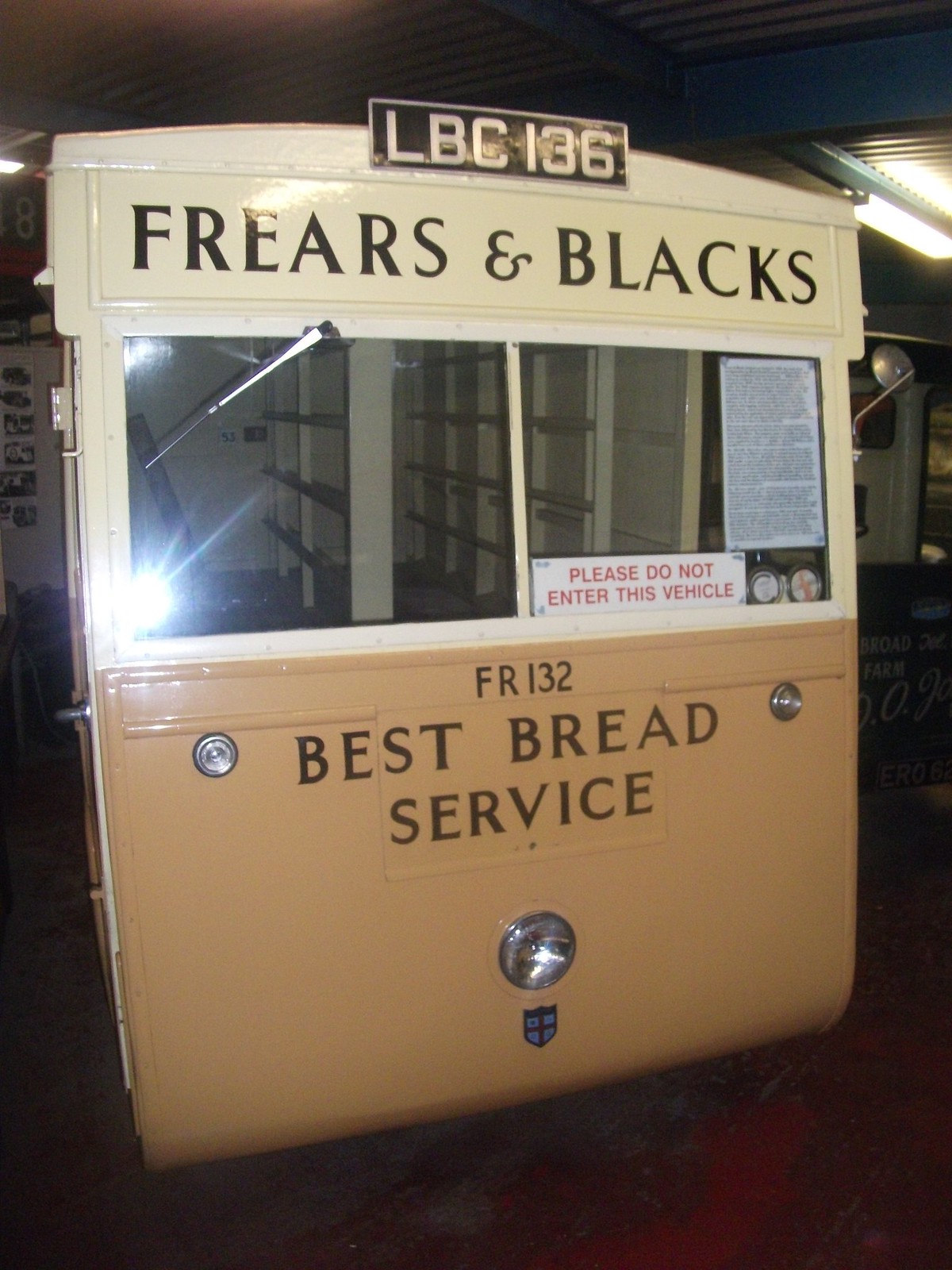The photograph captures the front part of a vintage, cream and brown vehicle with a distinctly square design, likely displayed indoors at a museum. The vehicle's roof is slightly rounded, and it prominently features a rectangular license plate at the top with the text "LBC 136" in white on a black background. Below this, on the cream-colored section above the windshield, the name "Frears and Blacks" is written in black, all caps serif font. The windshield consists of two large square panes, the left one adorned with a silver metal window wiper, while the right window has a large piece of A4 paper covered in text. A clear red and white sign on the windshield warns, "PLEASE DO NOT ENTER THIS VEHICLE."

Below the windshield, the lower light brown section of the vehicle displays "FR 132" and the phrase "BEST BREAD SERVICE" in centered, all caps black text. Flanking this text are two small lights, with an additional smaller light situated in the center at the bottom. Beneath this light is a blue and black shield emblem.

The background suggests an indoor exhibit, with white walls and a blue and white ceiling. Yellow lights illuminate the space, and there are trolleys and various objects, including another sign displaying "Broad Farm." A notable detail is the fluorescent-colored lighting at the top right corner, adding a modern touch to the otherwise retro scene. The floor beneath the vehicle is a blend of red and gray hues.